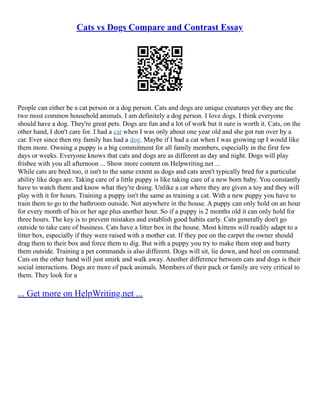The image features a page from an essay titled "Cats vs Dogs: Compare and Contrast Essay" against a white background. The title, prominently displayed at the top, is underlined. Directly below the title is a centrally placed blue and underlined hyperlink alongside a QR code. The essay discusses the author's preference for dogs over cats while reflecting on personal experiences. The text mentions that people can either be cat or dog enthusiasts, highlighting that both animals, despite being unique, are the most common household pets. The author recounts their fondness for dogs, describing them as fun yet challenging to care for, and laments a childhood incident involving a cat. The essay is written in a font resembling Times New Roman. The bottom of the page contains another blue, underlined hyperlink that directs readers to "get more help on helpwriting.net."